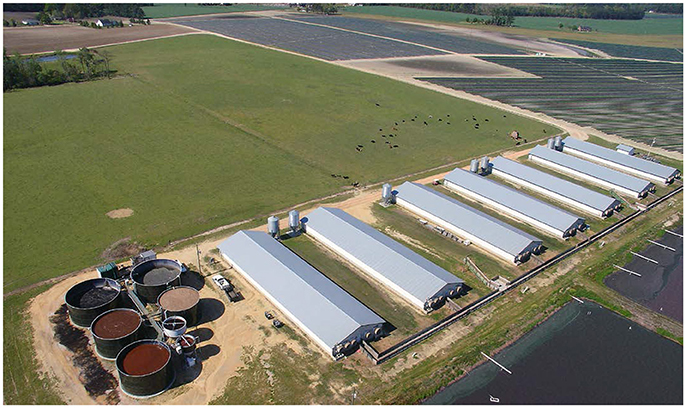This aerial photograph, likely captured by a drone, showcases a sprawling processing plant. The focal point of the image consists of seven large, elongated white buildings reminiscent of barns, organized in a staggered manner towards the right side. Adjacent to these buildings on the lower left is a sizable tank farm, featuring numerous cylindrical tanks. Directly to the right of the buildings lies a parking lot, while a vast green field spans the upper center of the image. Overhead, birds can be seen, adding a dynamic element to the scene. In the lower right corner, there’s a pond, suggesting the presence of water management within the facility. A distinctive feature is the long covered walkway attached to the leftmost building, connecting all the barns as it extends towards the right, indicating a well-integrated infrastructure within the complex.